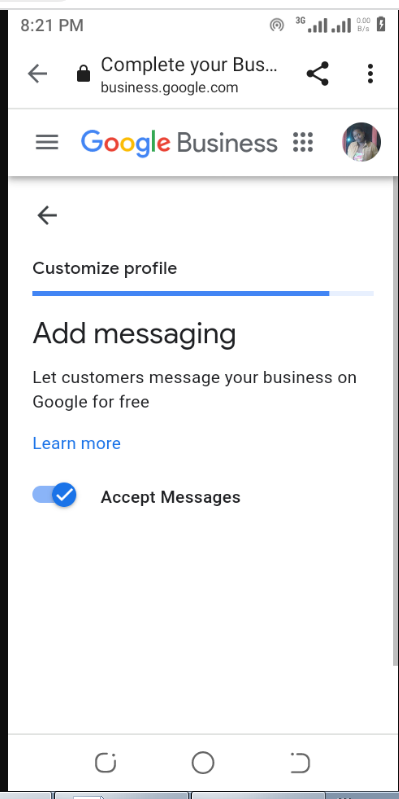The screenshot displays a Google Business profile on a smartphone screen, timestamped at 8:21 PM, with a 3G network signal and full battery. At the top of the screen, there are two network indicators, suggesting the presence of dual SIM functionality.

Centered on the screen are the words "Complete Your Business," with a lock icon and a left-pointing arrow on the left, indicating the profile is currently locked. To the right of this phrase, there is a share icon followed by three vertical dots for more options. Below this section appears the URL "Business.Google.com."

A row featuring three horizontal bars sits beneath this header, followed by the colorful Google Business logo in the center, nine dots representing various Google business applications, and a profile picture of a woman. An arrow pointing left appears below this row, alongside the text "Customize Profile," indicating the option to customize the profile with a progress bar below it showing 90% completion.

Further down, bold text reads "Add Messaging," with smaller text below offering the option for customers to message the business on Google for free. This includes a "Learn More" link and the selectable option to "Accept Messages," which has already been activated in this screenshot.